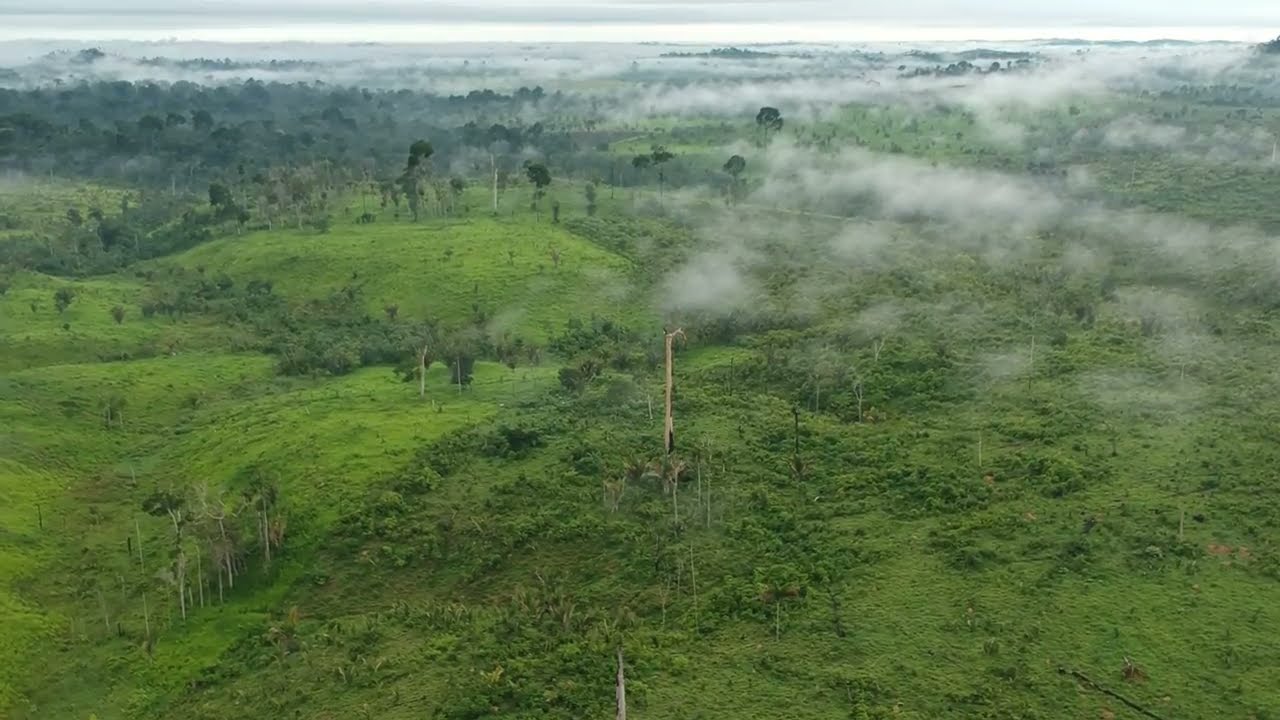The image showcases a lush, verdant landscape, predominantly covered in light green grass with occasional patches of darker green. The scenery extends into rolling hills that dominate the foreground and middle ground. Scattered throughout are very thin, short trees and clusters of green bushes. More prominent in the background are dense formations of dark green trees, appearing thicker and more closely packed together.

A notable feature of the scene is the mist or fog, which blankets parts of the landscape, particularly in the upper right and background areas. This light white mist creates an almost ethereal atmosphere, blending with the horizon that seems to stretch indefinitely. The sky is overcast, contributing to the overall soft light of the daytime image, casting a grayish hue that accentuates the lushness of the vegetation.

Bare trees without leaves are visible in the foreground, juxtaposed against the backdrop of dense greenery. Small brown patches of grass and dark brown dirt clumps are sporadically dispersed, adding to the natural diversity of the terrain. This higher vantage point offers a panoramic view, giving a sense of the expansive wilderness devoid of buildings, people, or animals.